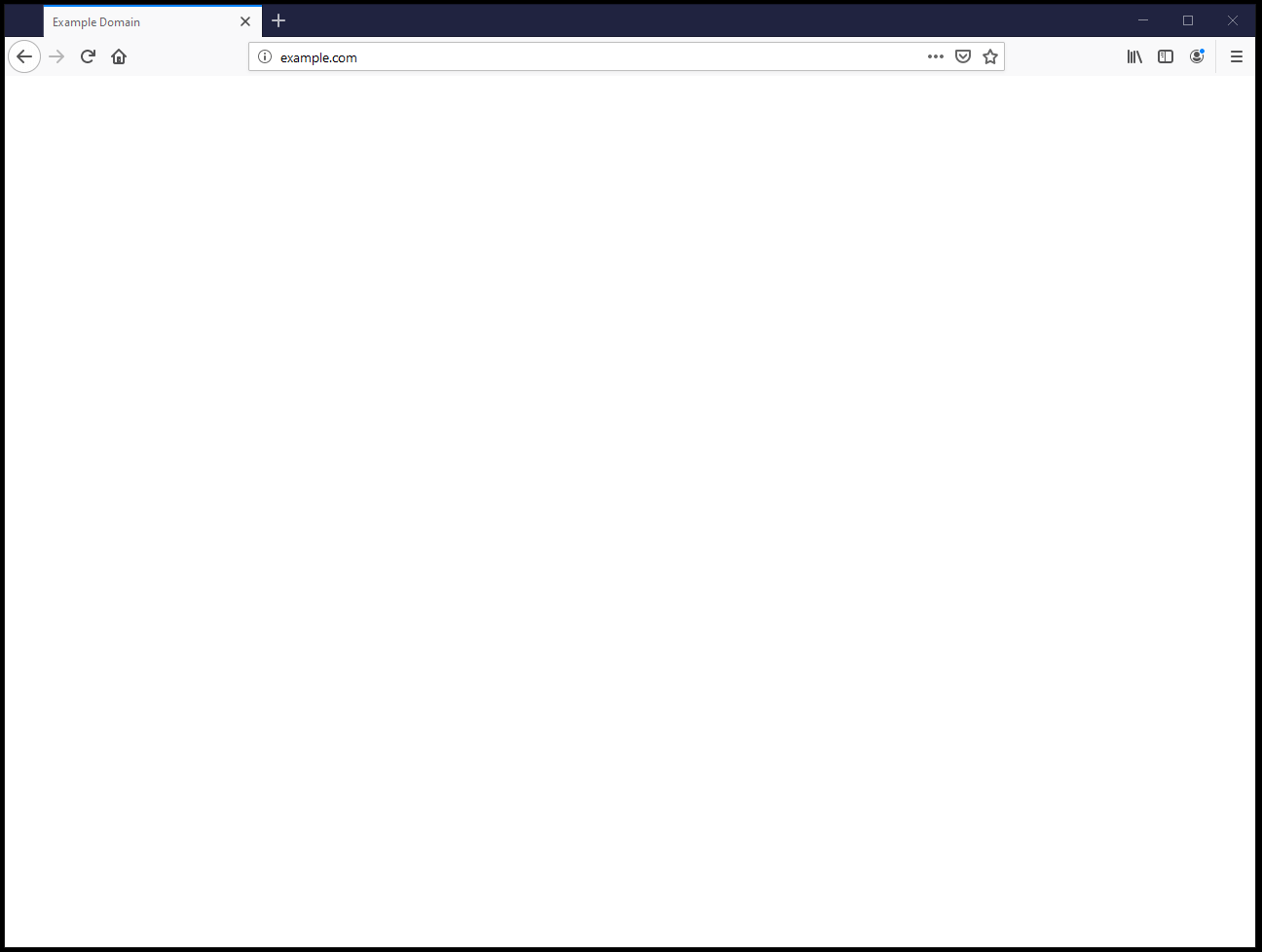A screenshot depicts a web browser interface on a white background. At the top, a new tab button marked with a plus sign, a square icon with a dash, and a close (X) button are visible. Navigation buttons are situated full left to right, including a left arrow, a right arrow, and a refresh button, followed by a home icon. 

In the address bar, the URL "example.com" is prominently displayed next to a circular icon featuring an eye, indicating a privacy or view option. Adjacent to the URL, a badge and a star icon are present, possibly for bookmarking or indicating a special status. Also present are three small stars which might represent a rating or security status. On the far right of the address bar, a stack of books icon and two rectangle icons are seen, most likely shortcuts to different functions or bookmarks.

Further, a profile icon with a blue circular badge, denoting either an active session or notifications, and a hamburger menu icon, signifying additional options, complete the browser's toolbar.